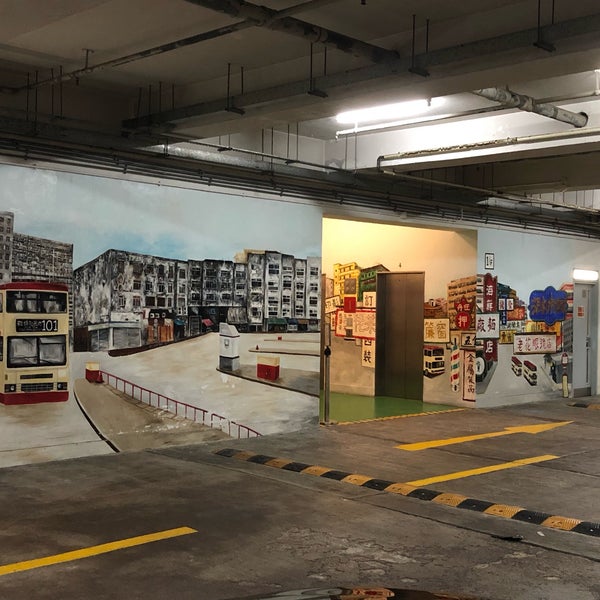The image is a color photograph in a square format featuring a detailed mural on the wall of an underground garage structure. The foreground showcases an asphalt parking lot marked with yellow directional arrows pointing in both directions, a black and yellow striped speed bump running diagonally from the upper left to the bottom right, and a series of lights on the ceiling. 

The wall mural itself spans a single story in height and consists of several distinct sections. On the left side, there is a vivid painting of a yellow double-decker bus with red accents, facing the viewer. This bus stands against a backdrop of gray buildings, which seem abandoned and dilapidated. The scene also includes a small red metal fence separating the bus from an imaginary sidewalk. 

In the center of the mural, there's an actual entrance that reveals a view into the hallway leading to an elevator, marked by a vertical black door and a green floor. To the right of this entrance, the mural continues with depictions of more buses, lanes, and buildings, maintaining a similar style that merges representationalism and realism. The overall artistic treatment is very detailed, making the paintings a striking visual element within the otherwise functional space of the garage.